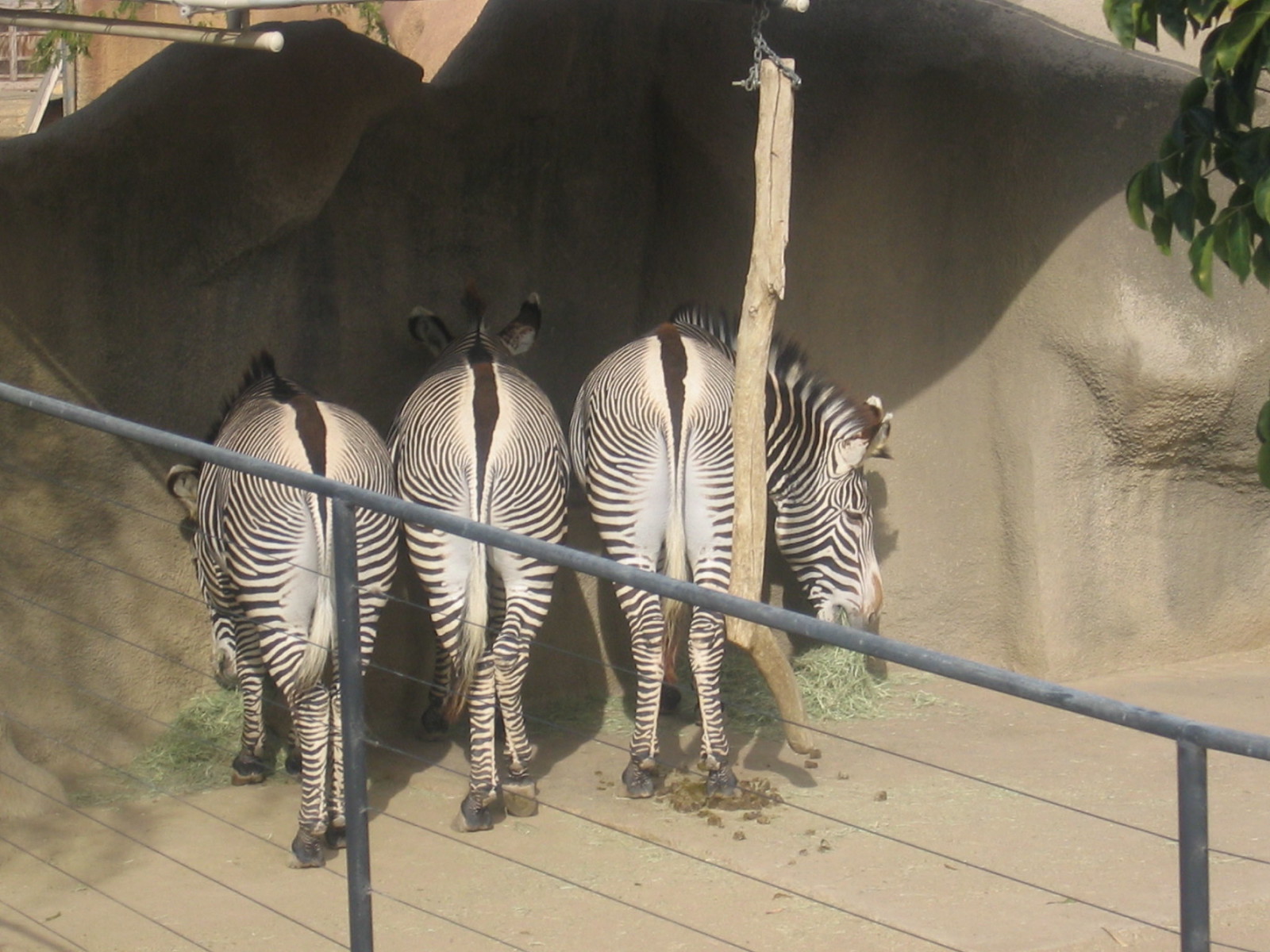This landscape-oriented color photograph shows a zoo habitat featuring three zebras, seen from behind metal railings composed of a top bar and multiple thinner horizontal bars. The zebras, primarily positioned in the central part of the image, are grazing on greenish hay-like grass near an artificial cave structure. The zebras' stripes are white paired with darker, deeper brown hues rather than the traditional black. The middle zebra's head is obscured, while the right zebra bends its neck slightly to the right, revealing a partial view of its head. The left zebra's head is only subtly visible. The top right-hand corner of the photograph features green leaves from a nearby tree, adding a touch of natural greenery, while the upper left side includes a bar and possibly some stairs, part of the broader habitat setting. Visible in the habitat foreground is some of the animals' defecation, providing a candid glimpse into their daily life.